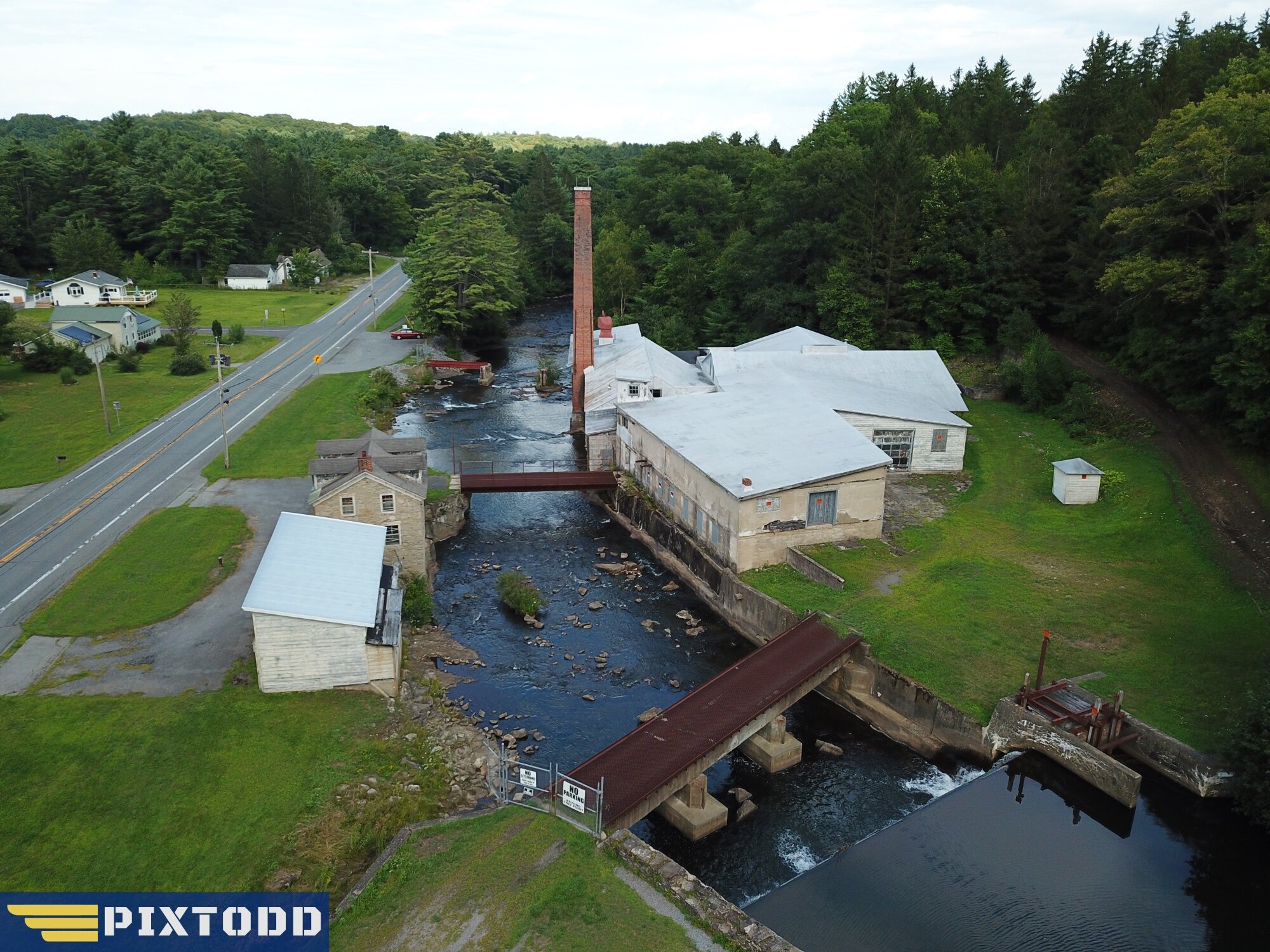The overhead drone shot captures a residential area dominated by a dark, flowing river that runs through its center. Small brown footbridges dot the river, connecting paths to various beat-up houses with slanted roofs, seemingly designed to drain water directly into the river. This scene appears to be in the late afternoon, with the sunlight softly illuminating the area.

On the left side of the image, a two-lane road, flanked by electric and light poles, extends from the middle to the top of the frame. The right side is marked by green grassy lawns and fields, with occasional small buildings. Surrounding the entire area are dense clusters of large, lush green trees and patches of greenery.

In the middle of the image, a towering brown chimney rises prominently above the area, suggesting an industrial environment. A mix of residential and possibly industrial buildings with triangular roofs and lawns is visible on either side of the river. At the bottom left corner, a logo featuring three yellow lines and some text that reads "Mix Todd" can be seen, although partly obscured. The sky overhead is light powder blue with scattered white clouds, adding to the serene yet somewhat worn appearance of the town.